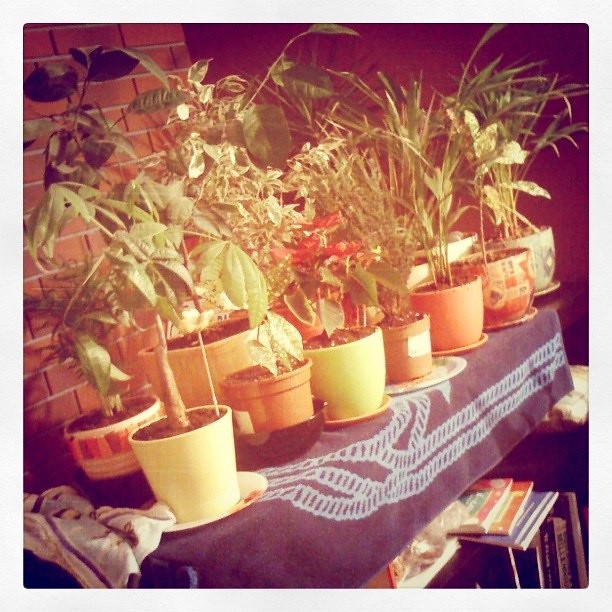This image is a sepia-toned photograph, possibly filtered for an aged effect, featuring a collection of approximately a dozen potted plants. The plants, mostly green with one featuring red flowers, are placed on a blue tablecloth with light blue line designs. The tablecloth covers a table set against a reddish-brown brick wall. Each plant is in a similarly sized pot, with some variations. Below the table, there is a mix of books and magazines, some stacked horizontally and others standing vertically. The scene exhibits a cozy indoor setting with an aesthetic reminiscent of an old, filtered photograph.